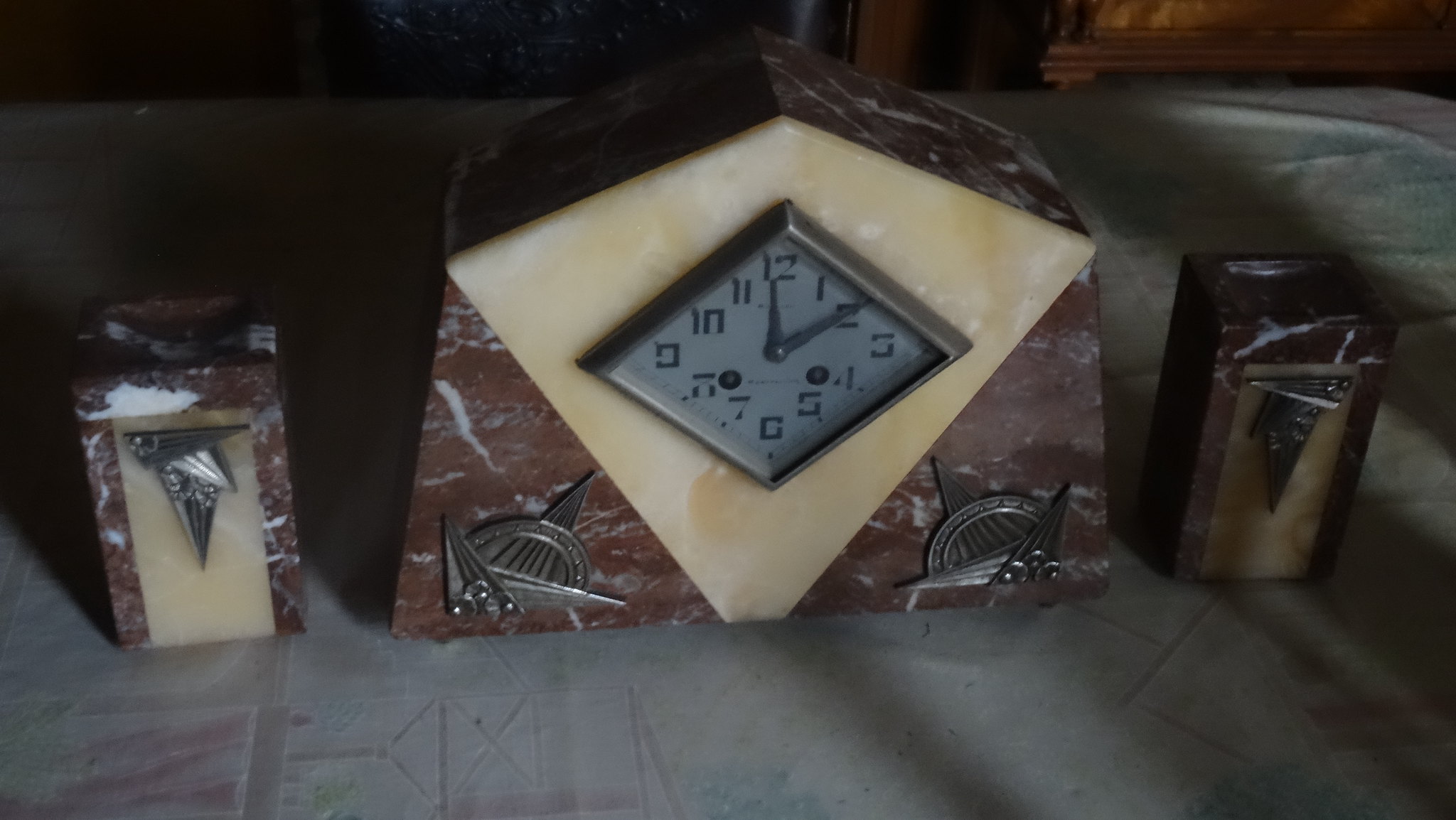This indoor photograph features an ornate and elaborate desk set centered around a visually striking marble clock. The clock itself is primarily made of contrasting brown and white marble, arranged in triangular shapes at the bottom corners, while the top section showcases a diamond-shaped cream-colored material, possibly mother of pearl. The clock face is diamond-shaped, framed in black metal with traditional numbered dials that read ten past twelve. Noteworthy are the intricate metal inlays at the bottom corners of the clock, depicting what appear to be insignias with wings, sails, or an arched dome. Flanking the clock are two similarly designed square-based pen or pencil holders, constructed from the same two-tone marble and lighter material, featuring the same metal insignias. All pieces rest on a table covered with a white-patterned tablecloth with subtle pastel streaks, situated in a darkened area where shadows accentuate the elegance and intricate details of the desk set.